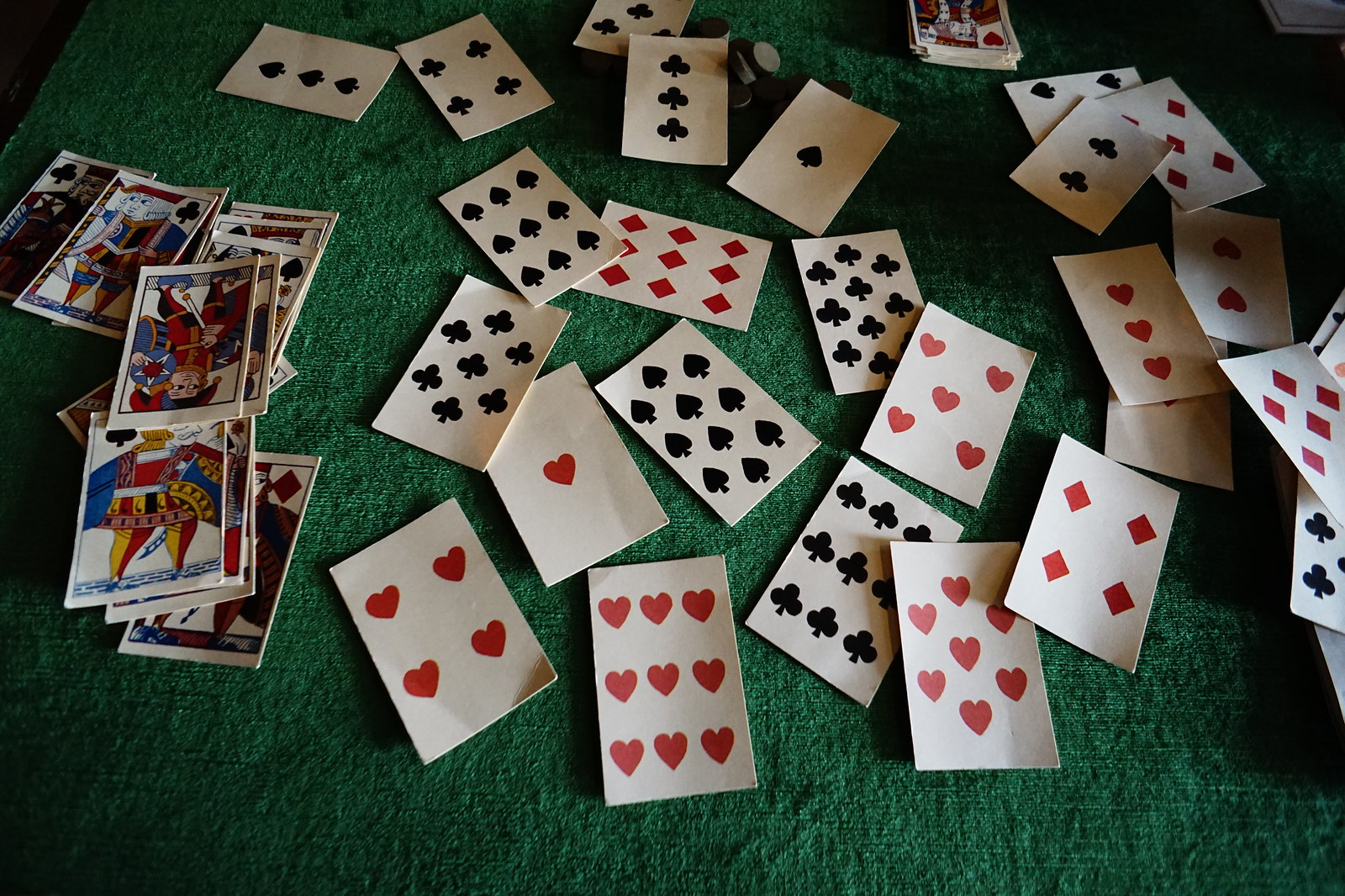The image presents a vividly detailed scene of playing cards scattered across a green surface. The green background dominates the entire image with the exception of the top left corner where a speck of brown is visible. Also in the top left corner is a small snippet of a white piece of paper adorned with a black trim, peeking modestly into view.

To the left side, there's an elaborate arrangement of playing cards, primarily showcasing the face cards—Jacks, Queens, and Kings from various suits. This heap extends about an inch from the left edge, spanning roughly a third of the image's width and reaching about two inches up from the bottom before looping back to the left edge. Among the prominent face cards, you can spot the Jack of Clubs and the King of Clubs, as well as the Jack of Diamonds, totaling around twelve face cards visible on the surface, with the remaining ones concealed beneath.

In the top left pile, adjacent to the reveal of the white paper, you can detect half of several card faces stacked. The top card in this cluster is a Jack of Hearts. These cards lack numerical indices, instead displaying symbols correlating to their rank, such as nine hearts for the Nine of Hearts and three diamonds for the Three of Diamonds. Included in this assortment are the Three of Spades, Four of Clubs, Five of Clubs, Three of Clubs, Ace of Spades, Three of Clubs again, Four of Diamonds, and Five of Diamonds, layered chaotically.

In the center of the image, the cards are more dispersed, offering a clear view of various cards. Prominently displayed are all the Nines grouped together with an Eight and an Ace positioned beneath. Two Nine of Spades cards appear slightly hidden behind a Ten of Spades.

On the right side, towards the middle, there's a smaller stack of four cards. The top card here is the Ten of Diamonds, with a club card visible below it, followed by two more cards—one red and one black—partially extending off the page.

This visually intricate arrangement produces a striking tableau of randomness and order, displaying the diversity and beauty of a deck of playing cards.